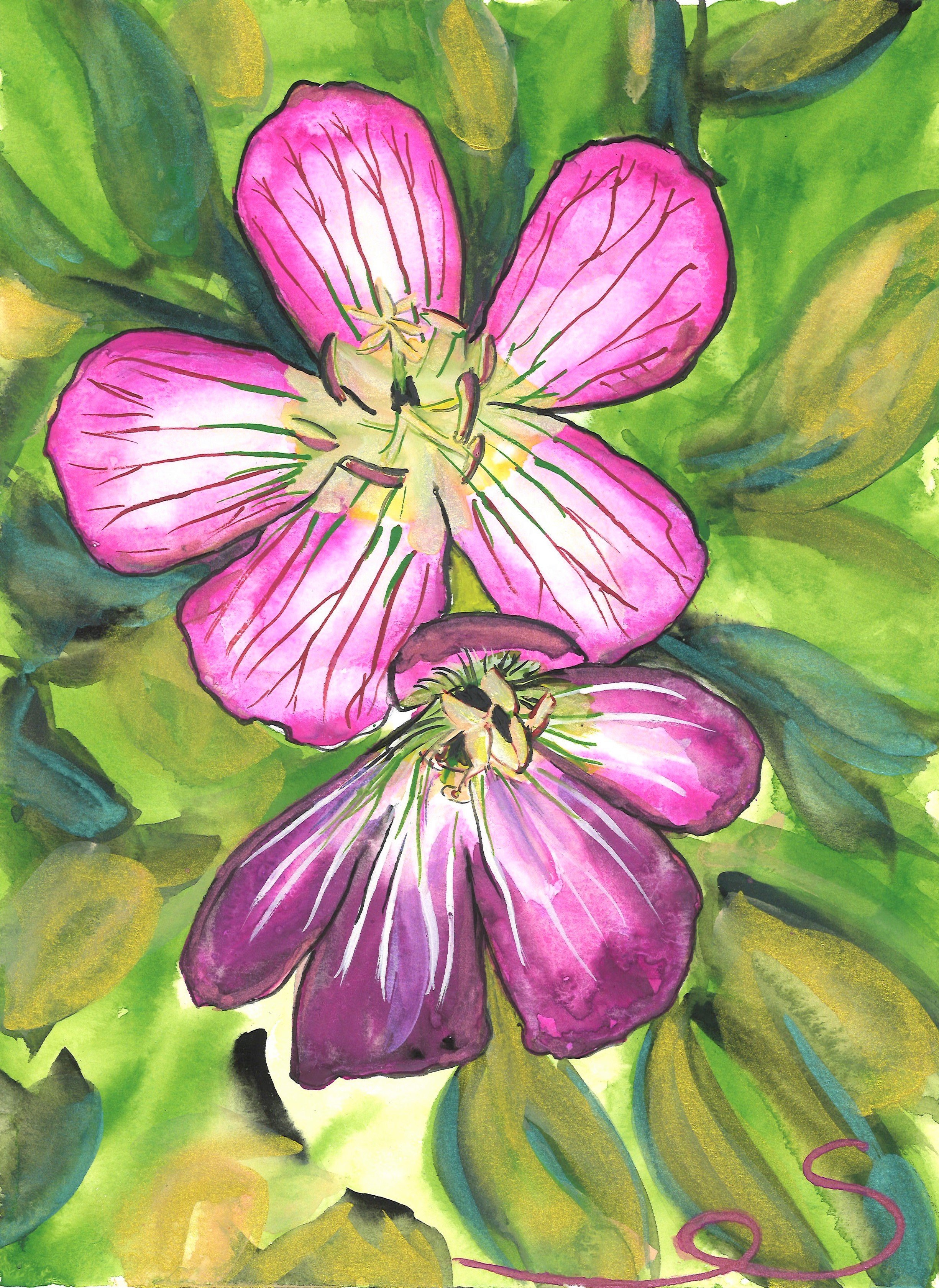This vividly colored artwork, likely a watercolor or gouache painting, features a rich and vibrant portrayal of flowers and leaves. The painting, in a portrait orientation, captures a lush, abstract background with varying shades of green ranging from deep and dark to bright and dull, along with hints of yellow and dark brown for contrast. Centered in this verdant setting, there are two prominent flowers: the top flower is widely open, displaying purplish pink petals adorned with red and white veining, and a yellow center. Below, a slightly closed flower exhibits similar purplish pink petals with striking white stripes and a yellow-green center. The bottom edge of the painting features an artist's signature, resembling a swirl or an 'S', crafted in the same accent pinkish-purple hue as the flowers. This signature adds a personal touch to the exquisitely detailed, abstract composition.